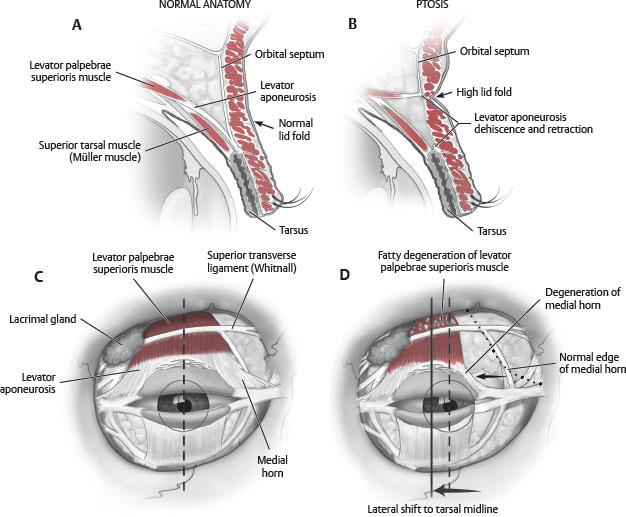The diagram from the anatomy book is divided into four quadrants labeled A, B, C, and D. Quadrant A, at the top left, displays normal eye anatomy, specifically highlighting the levator palpebrae superior muscle. Just to the right, quadrant B is focused on ptosis and marks features such as the orbital septum. In the bottom left, quadrant C contains a detailed illustration of the human eye, showcasing various glands and muscles, including labels for the medial horn and normal structures like the superior tarsal muscle. Lastly, quadrant D, positioned at the bottom right, presents an eye affected by ptosis, indicating issues such as the degeneration of the medial horn, a high lid fold, and fatty degeneration. Both bottom quadrants offer head-on views of the eye with extensive labeling of muscles, glands, and anatomical changes associated with ptosis.